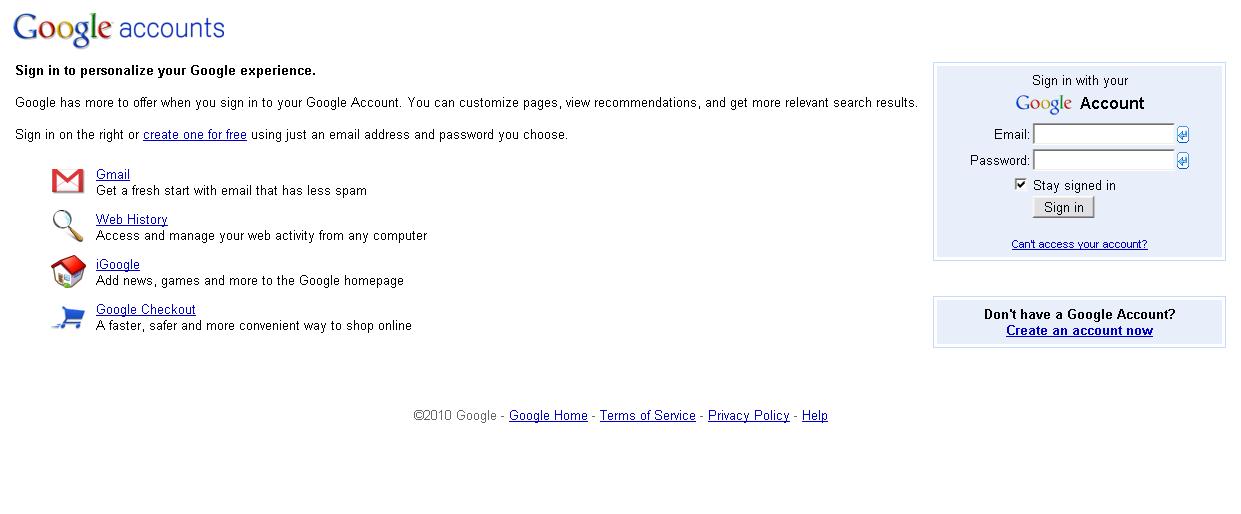The image showcases the familiar Google search homepage. Dominating the top, the classic Google logo is displayed in its iconic blue, red, yellow, and green lettering. Beneath this vibrant logo, the text reads "Google Accounts," and it is followed by the tagline: "Sign in to personalize your Google experience."

The image emphasizes the benefits of signing into a Google account. It states users can customize their pages, receive tailored recommendations, and enjoy more relevant search results. A prompt on the right encourages viewers to either sign in or create a Google account, which can be done for free using a chosen email address and password.

Below this main section, a series of promotional features are displayed:

1. **Gmail**: The caption highlights the efficiency of Google's email service, particularly its capability to block spam, promoting a "fresh start" with cleaner inboxes.

2. **Web History**: This feature offers users the ability to access and manage their web activities from any computer, ensuring seamless continuity across devices.

3. **iGoogle**: A customizable homepage where users can add news, games, and other personalized content.

4. **Google Checkout**: Introduced as a faster, safer, and more convenient way to shop online, enhancing the e-commerce experience.

On the right-hand side of the image, there is an explicit sign-in area for Google accounts, supporting users in accessing the full suite of personalized services.